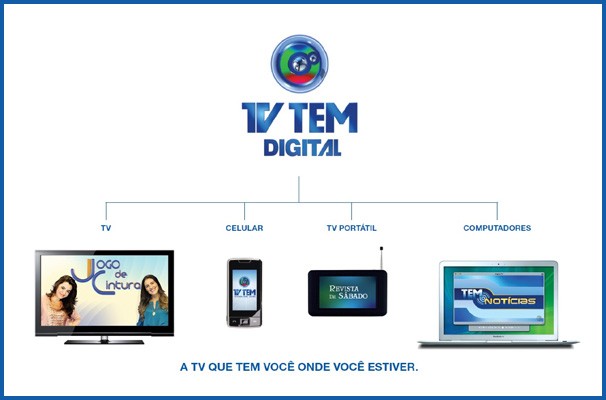The image is a rectangular advertisement with a thin navy blue border surrounding a white background. At the top center, there is a circular logo incorporating the colors red, green, and blue. Below the logo, the words "TV TEM digital" are prominently displayed in blue text. A flowchart extends downward from the logo, dividing the image into sections. On the left, a line leads to the label "TV" above an image of a TV monitor. Moving right, the next section is labeled "cellular" with an image of a cellphone underneath. Further right, the label "TV portatil" is above an image of a small tablet. Finally, on the far right, the label "computadoras" is positioned above an image of a laptop. At the very bottom of the image, there is a line of text in a foreign language: "A TV QUE TEM VOCE ONDE VOCE ESTIVER." The predominant colors in the image include blue, white, green, red, light blue, gray, and black. This advertisement appears to be styled as a poster or sign and is likely intended for a different language-speaking audience.